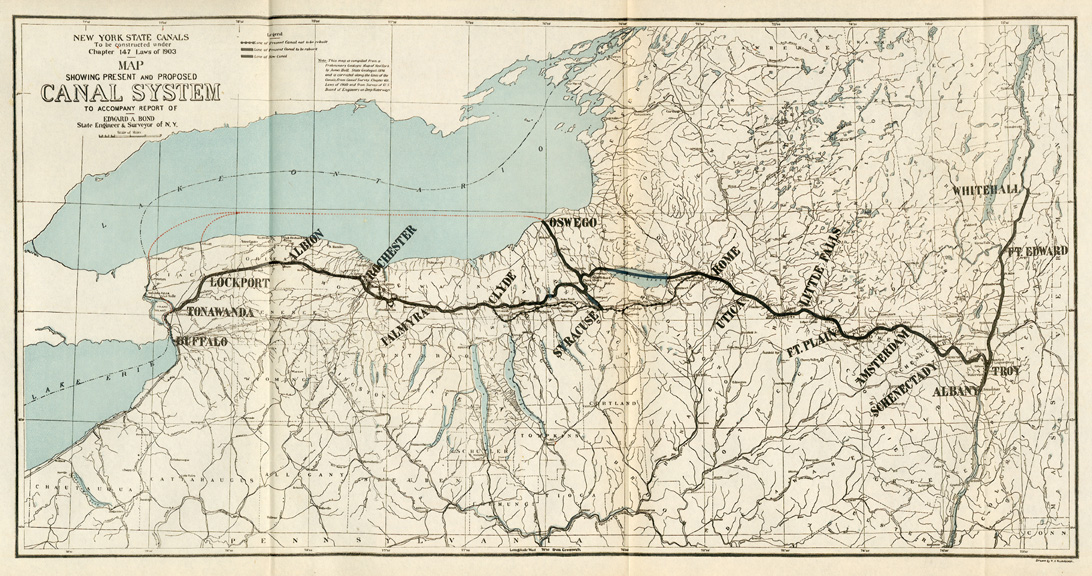An antique map labeled "New York State Canals to be Constructed under Chapter 147 Laws of 1903" accompanies a report by Edward A. Bond, State Engineer and Surveyor of New York. The map, depicting the proposed and present canal systems in New York State, appears aged and weathered. In the top left corner, it mentions the canal system, specifically detailing the connection between the Hudson River and the Great Lakes. Principal towns along the black line representing the canal route include Buffalo, Tonawanda, Lockport, Albion, Rochester, Palmyra, Clyde, Syracuse, Oswego, Rome, Utica, Little Falls, Amsterdam, Schenectady, Albany, Troy, Fort Edward, and Whitehall. The map's detailed depiction extends from Lake Erie and Lake Ontario in the west to the various towns and the river to the east, reflecting a comprehensive network aimed at linking the waterways across the state.